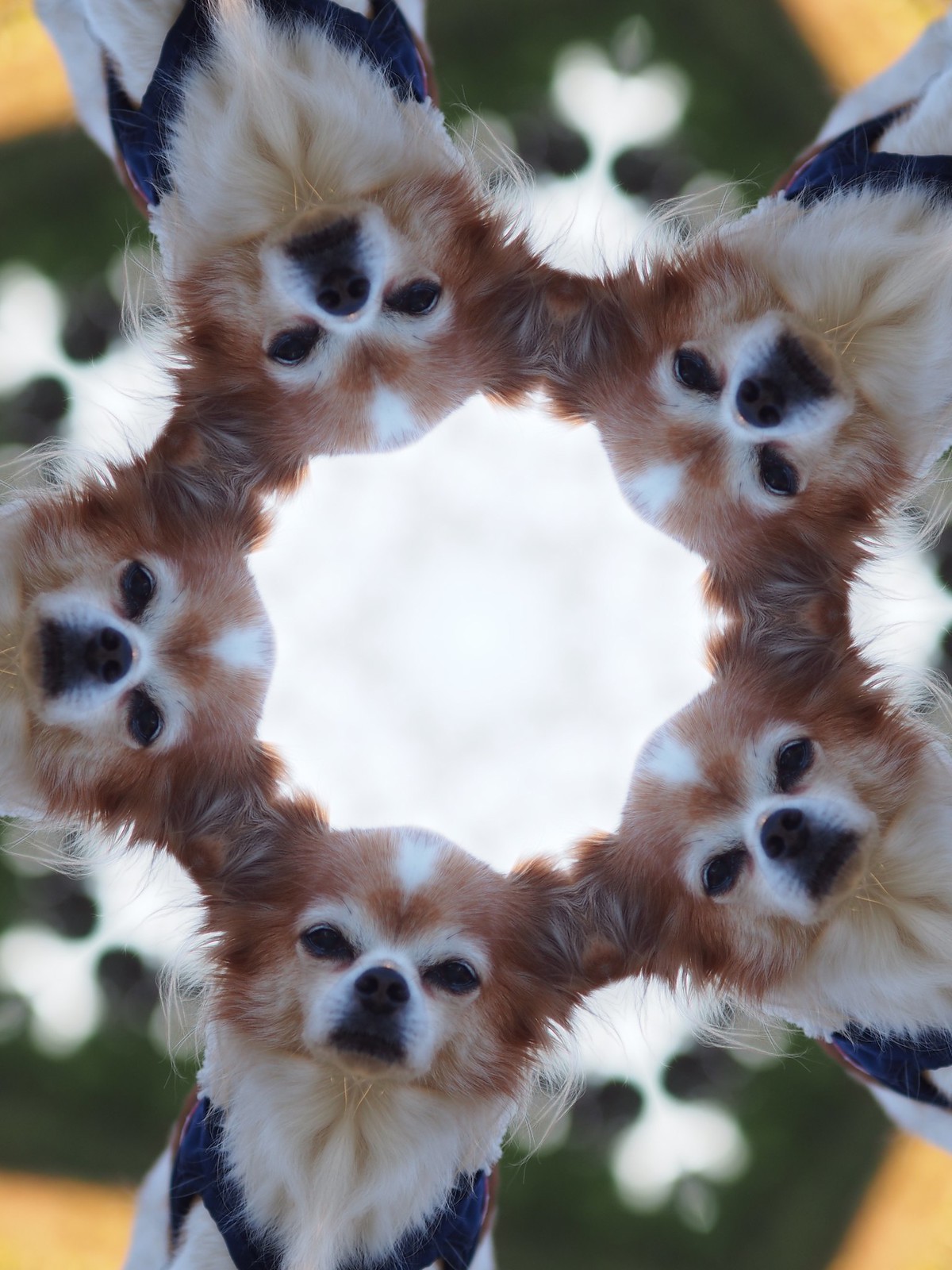A mesmerizing, kaleidoscopic image captures the essence of an outdoor setting with a charming, small dog at its heart. The photograph has been artistically edited to create a circular, mirrored design, featuring five identical images of the dog, each iteration forming a seamless loop with their ears touching to create a continuous circle. The background between each dog displays a blend of green and yellow, suggesting the presence of trees or foliage.

The dog, possibly a chihuahua mix, is distinguished by its reddish-brown fur accented with a white triangle on its forehead, white patches around the eyes, muzzle, and a white ruff. It has a black nose, dark eyes, and a black triangular area beneath the nose. The dog, dressed in a blue harness or jacket, appears older, with some graying around its face, giving it a wise, endearing look. The composition features a swirled, heart-shaped design of green behind the dog, adding to the artistic flair, and a red star-shaped space in the center where the heads converge. This creates an illusion as if the viewer is looking up at the dogs, all staring down intently and seriously. The interplay of colors and patterns results in a visually compelling and detailed depiction of this cute, little dog's image.